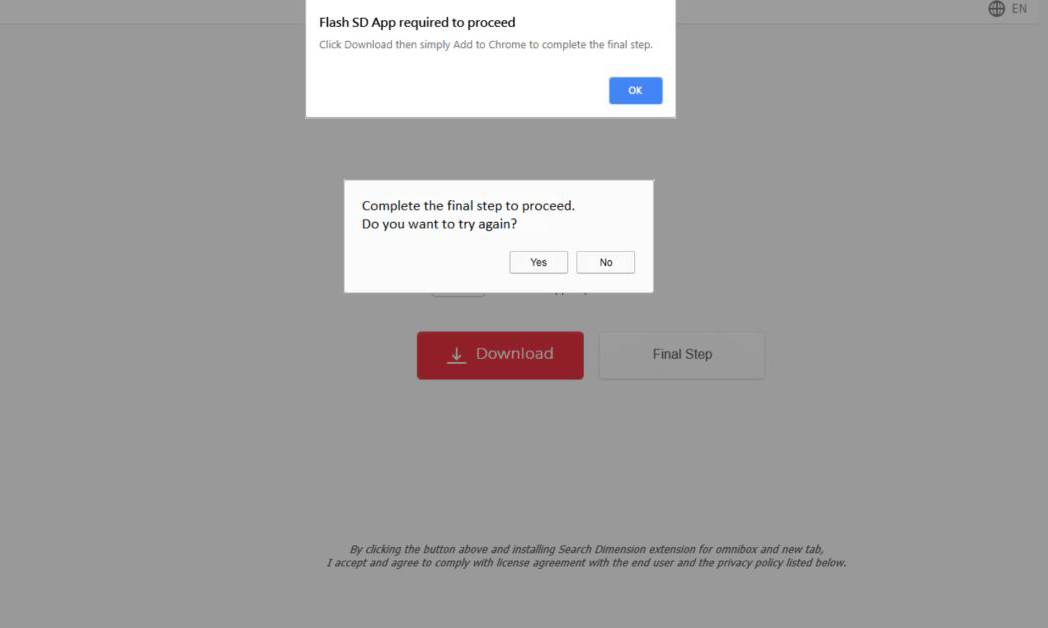The image showcases a web page filled with multiple pop-up messages and interactive buttons. The primary pop-up message reads, "Flash SD app required to proceed. Click download, then simply add to Chrome to complete the final setup." Below this message is a prominent blue "OK" button. Another pop-up message says, "Complete the final step to proceed. Do you want to try again?" 

On the page, there is a distinctive red clickable button labeled "Download" and a white button marked "Final Step." At the bottom of the page, a disclaimer states: "By clicking the button above and installing search dimension extension for Omnivox and New Tab, I accept and agree to comply with the license agreement with the end user and the privacy policy listed below." In the top right corner, the selected language is set to English.

The overall layout resembles an Adobe Flash installer interface, characterized by the red "Download" button. Aside from the download button, the final step button, and the disclaimer at the bottom, the rest of the page is predominantly blank and white.